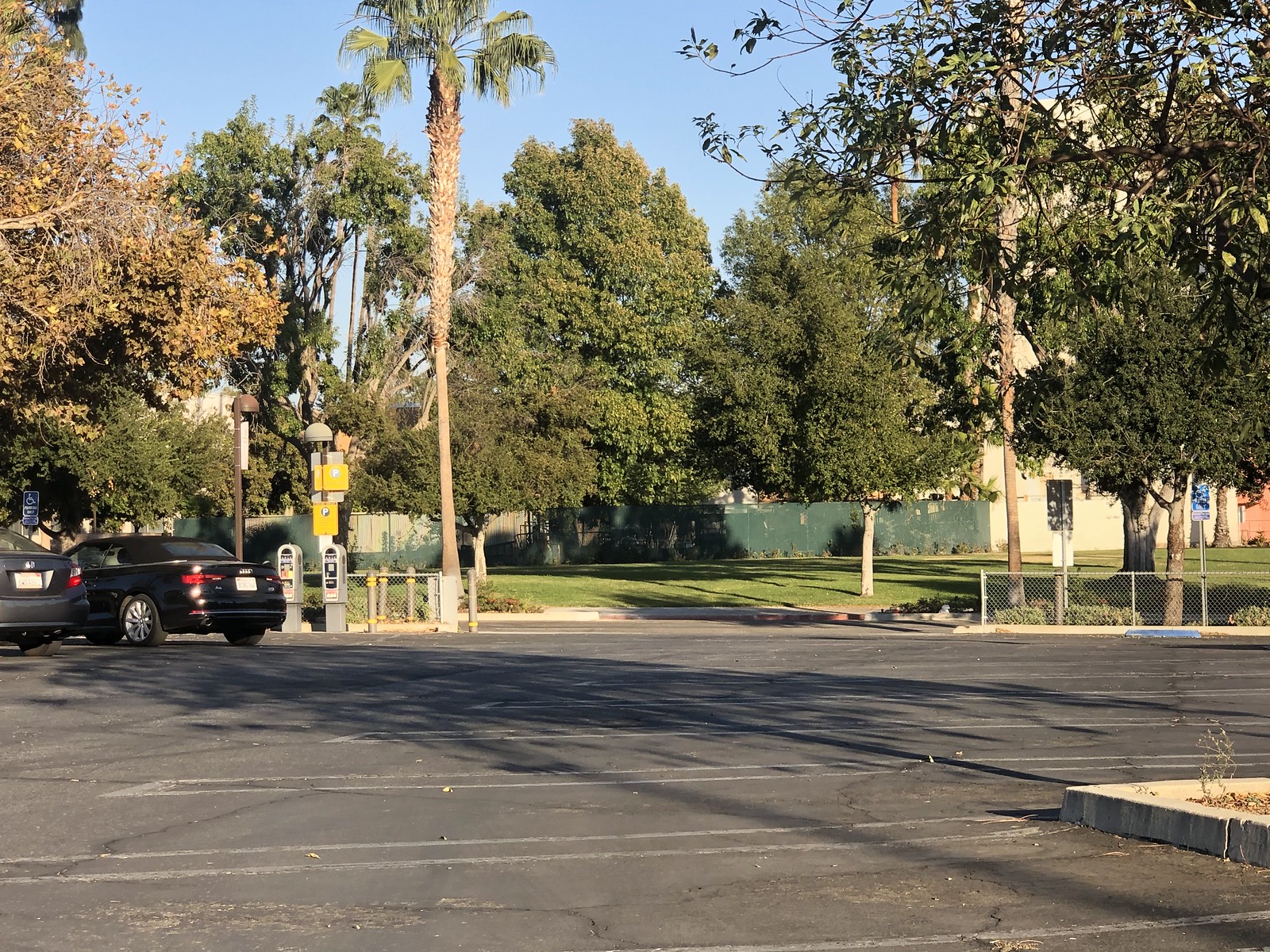A sunny day in what appears to be a somewhat neglected parking lot is captured in this photo. The blacktop exhibits visible signs of wear, with faded lines marking the parking spaces. In the distance, a chain-link fence with a green cover partially obscures the view, allowing only a subtle glimpse of what's behind it. Beyond the fence, lush green trees and grass frame a tan colored concrete building. Among the trees, one distinctly resembles a palm tree, while another shows signs of withering leaves. Two black cars are parked towards the back of the lot, though their models aren't discernible due to the distance. A potential area for parking meters or payment kiosks is vaguely visible further back. The clear blue sky casts shadows indicating that the photo was taken either during sunrise or sunset, though the exact position of the sun remains undetermined. The image lacks any noticeable text or additional subtle details.